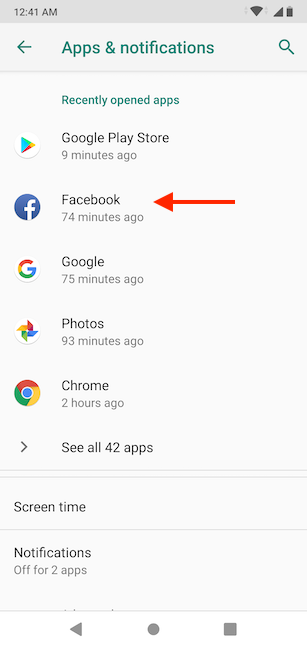A vertical shot taken at 12:41 a.m., likely captured on either a cell phone or tablet, displays the device's "Apps and Notifications" screen. The interface highlights the "Recently Opened Apps" section, listing Google Play Store, Facebook, Google Photos, and Chrome with respective usage times of 9 minutes, 74 minutes, 75 minutes, 93 minutes, and 2 minutes. There is an option to see all 42 apps, alongside an indicator showing notifications are turned off for 2 apps. Dominating the scene is a prominent horizontal red arrow on the right side, pointing left towards the Facebook icon, emphasizing the Facebook app which was last used 75 minutes ago.